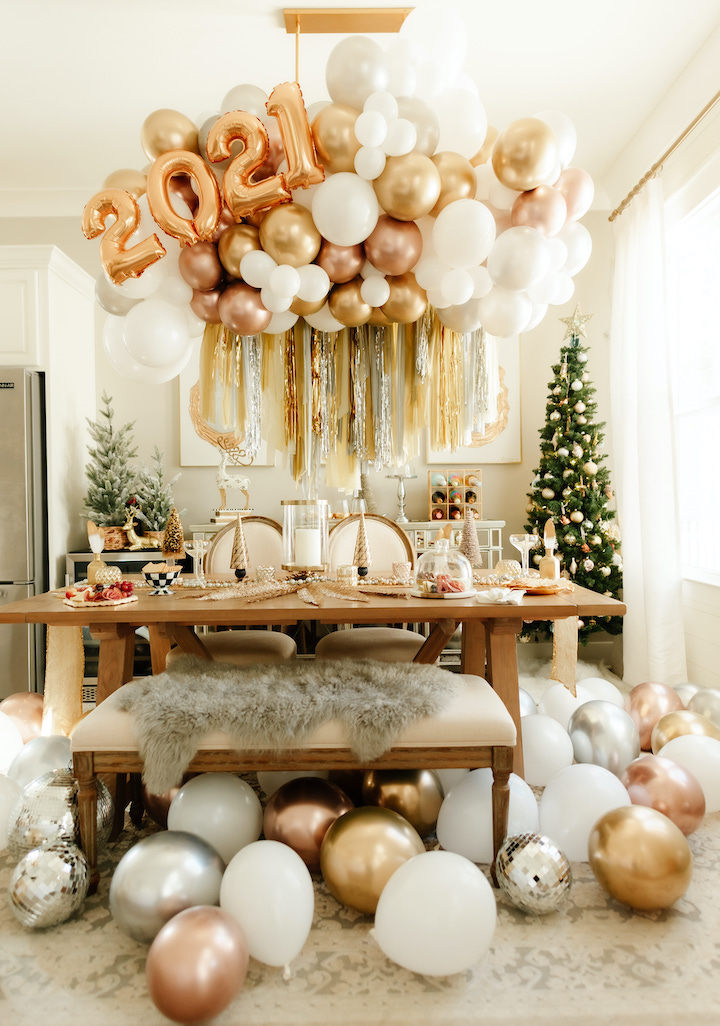The image portrays a dining room meticulously decorated for a New Year's Eve party in 2021, blending festive elements of Christmas and New Year celebrations. The room features white ceilings and walls with a grayish-green door to the left. Dominating the ceiling are clusters of gold, champagne, silver, and white balloons, with some streamers cascading down. Prominently displayed amidst the balloons is a large "2021" sign made from balloon numbers.

The room is accessorized with festive décor, including two Christmas trees: a fully decorated tree on the right with gold, silver, and white ornaments and a star topper, and an undecorated tree on the left. The back wall showcases abstract paintings featuring gold, silver, and bronze streaks, framed in gold. Beneath the paintings, a ledge holds various items such as Christmas balls, a plate on a spindle, and a reindeer sculpture.

The brown dining table is set with an elegant Christmas theme. It features two white chairs with gold borders and is adorned with mini gold Christmas trees, a large candle in a glass container with a gold top, candlesticks, and bowls containing fruit. Additionally, there are wine bottles on a rack and more decorative reindeer. A gray throw rug covers an ottoman, and the floor is dressed in a white and gray rug with scattered gold, silver, and white balloons. The overall aesthetic is gold-centric, creating a luxurious and festive atmosphere for the celebration.